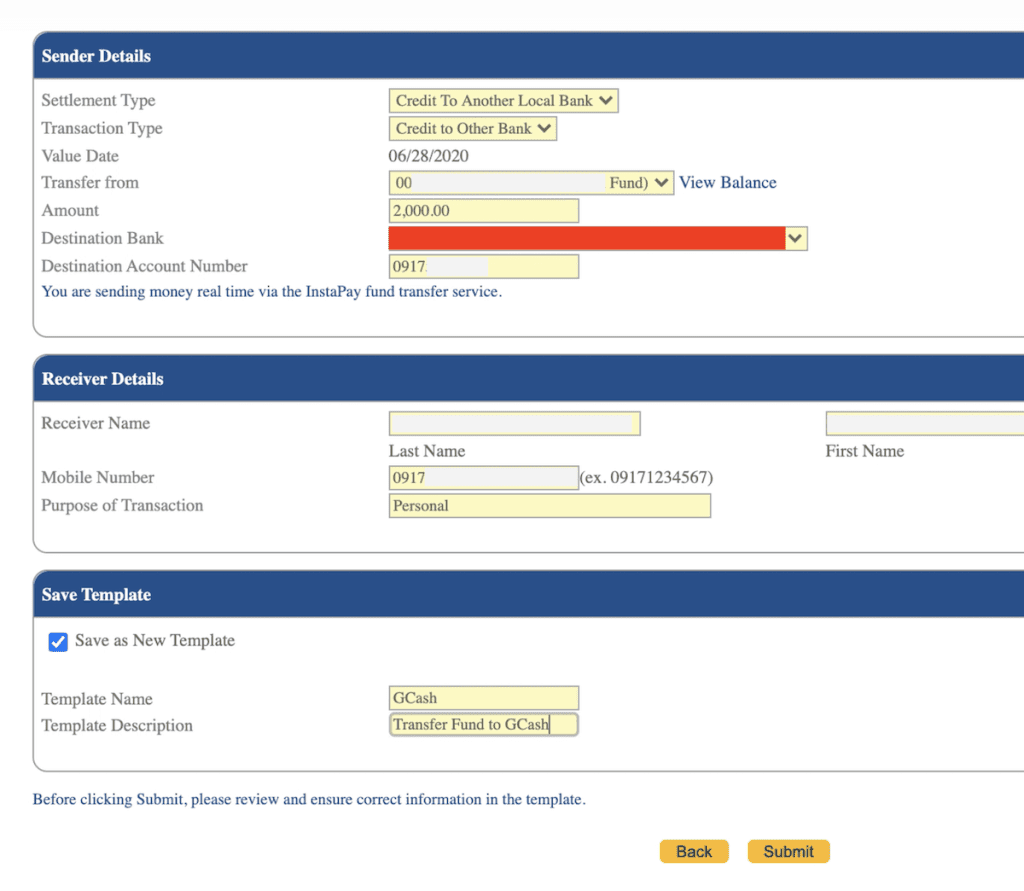The screenshot features an online form divided into three main sections, each clearly demarcated by horizontal blue bars. The top section is labeled "Sender's Details." It includes several fields designed for user input or selection:

1. Settlement Type
2. Transaction Type
3. Value Date
4. Transfer From Amount
5. Destination Bank
6. Destination Account Number

Below these fields is a note that reads: "You are sending money real-time via Instapay fund transfer service."

The middle section, marked by another blue bar, is dedicated to "Receiver Details." This section contains fields for:

1. Receiver Name
2. Mobile Number
3. Purpose of Transaction

The final section, also headed by a blue bar, focuses on saving the template. The top bar in this section reads "Save Template," followed by a blue box with a white checkmark labeled "Save as New Template." Below this are fields for "Template Name" and "Template Description." 

At the bottom of the screen, there's a cautionary instruction in blue text: "Before clicking submit, please review and ensure correct information in the template." This is followed by two orange buttons: one labeled "Back" and the other "Submit."